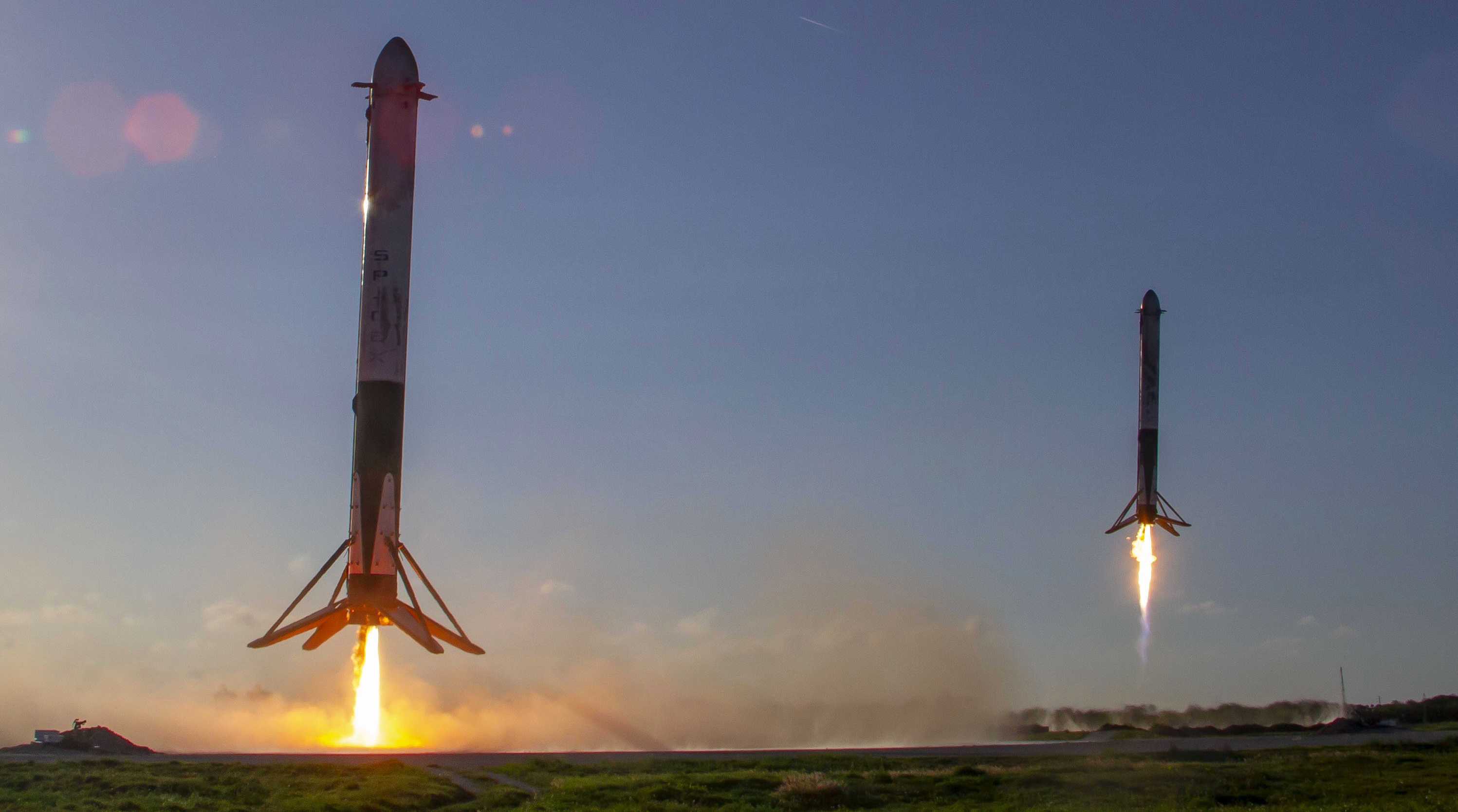This photograph captures a thrilling dual rocket liftoff. The scene unfolds on a vast, flat, grassy landscape with a small structure visible on the far left. Both rockets, emblazoned with the SpaceX logo in black lettering, dominate the image as they ascend into a mostly clear blue sky. The rocket on the right has ascended higher than its counterpart on the left, which, though closer to the viewer, has its fiery exhaust still scorching the earth below. Each rocket is a sleek, elongated cylinder featuring a rounded tip and painted primarily in white with red accents near the base, where red stabilizing fins are visible. Bright yellow and orange flames shoot out from the bottoms of both rockets, with swirling smoke adding to the dramatic effect. Additionally, a distant rocket stands upright but unlaunched on the right side of the frame, and overhead, a jet's contrail slices through the open sky. To the bottom left, a mound of dirt and a mechanical device, possibly for recording the liftoff, hint at the meticulous preparation behind this awe-inspiring event.